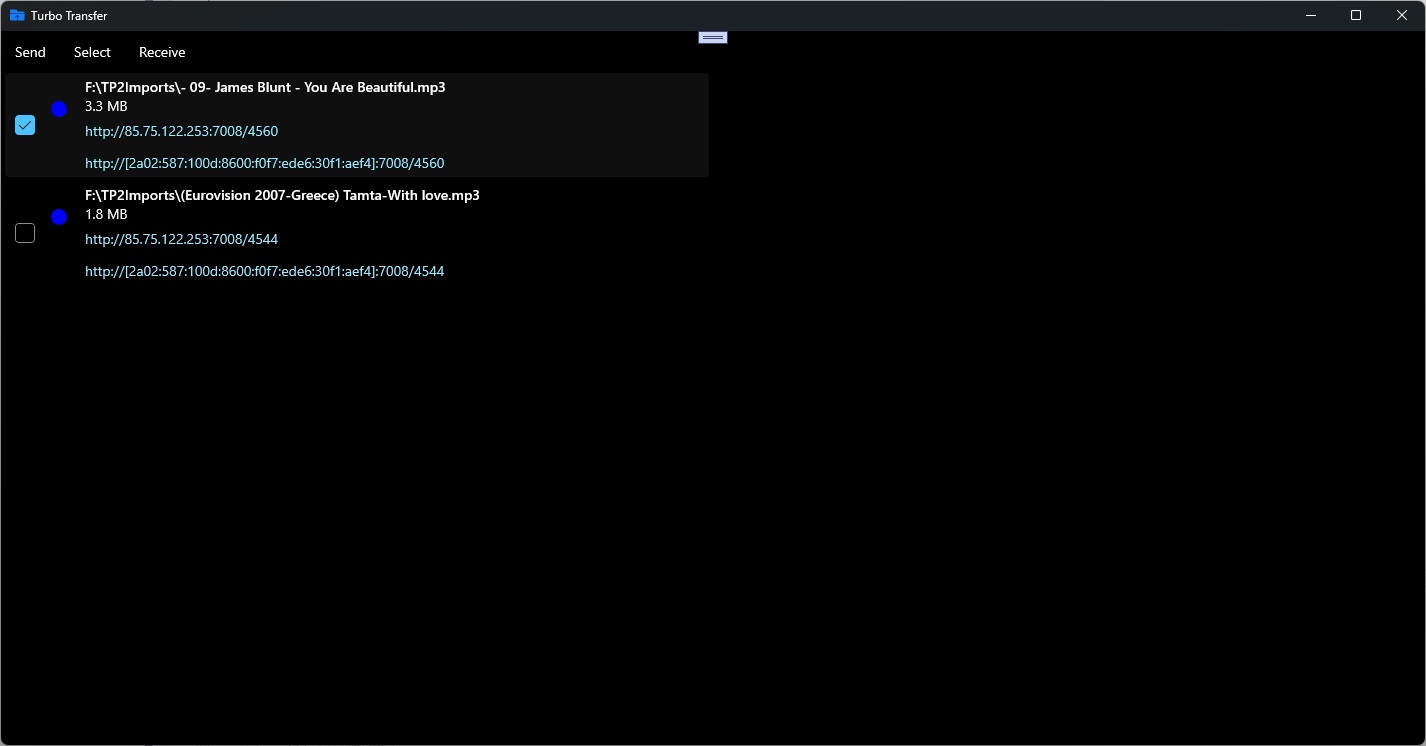This screenshot illustrates an interface from the TurboTransfer website, easily identified by its name featured in the upper left-hand corner. The website's design uses a black backdrop contrasted with white text, presenting files located on the F drive. An address displayed in light green text presumably represents the local host file or address.

Two files are listed in the interface: the first file named "ftmp2imports-09-jamesblunt-urbeautiful.mp3," a 3.3-megabyte MP3 file, has a check mark in its corresponding checkbox, indicating it is selected. The second file, identified as "f/http://tp2imports.eurovision2007-greeco.comta-withlove.mp3," has not been selected, as indicated by its unchecked box.

The visible toolbar offers three options—Send, Select, and Receive—providing functionality for managing the file transfers.